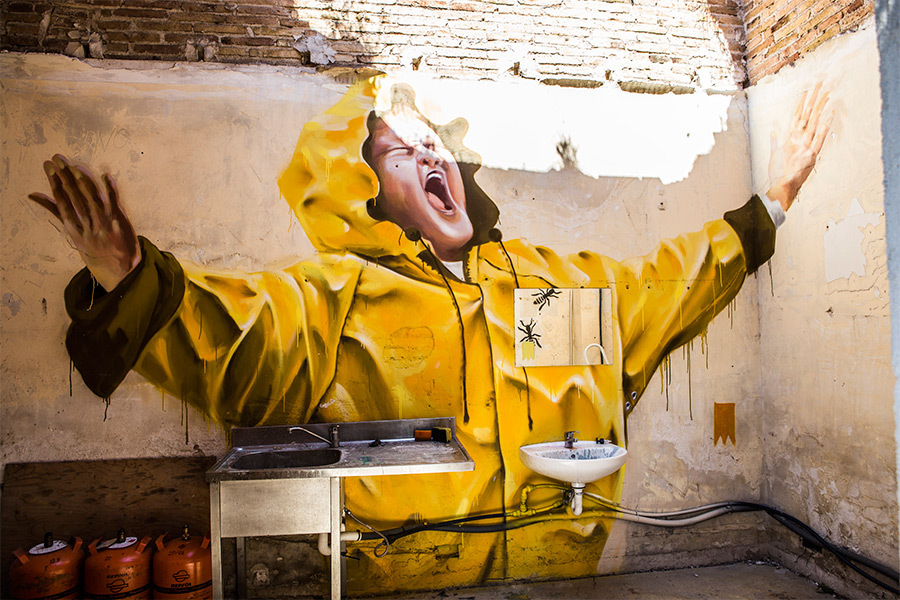The photograph captures a large, detailed mural set in a dank, industrial-like basement corner. The mural, spanning roughly 10 feet in height, depicts a young man in a yellow raincoat with his hood up, his arms outstretched to the sides, head tilted back, eyes closed, and mouth open, as if singing or making an appeal to the heavens. The character's interaction with the light streaming down from an opening in the ceiling emphasizes a divine or ethereal connection. This light source, possibly a sunroof or a hole in the roof, bathes the scene in a natural glow.

The mural is painted on a heavily cracked and stained white plaster wall, which covers the lower section. The upper part of the wall is composed of various rectangular brown bricks, their bare mortar lines clearly visible. Below the mural, the room contains a mix of elements including a small porcelain white hand sink, a stainless steel sink set into a somewhat unsupported metal counter, a mirror also marked with paint, and various pipes and wires strung along the walls.

In the lower left-hand corner of the photograph, there are three red or orange containers, possibly gasoline cans, equipped with spigots. Alongside the main figure in the mural, two small black ants are visible, crawling across a square painted on the raincoat, adding an intriguing touch to the artwork. The overall setting suggests a grimy, neglected space, yet the mural brings a vibrant, almost spiritual life to the scene.